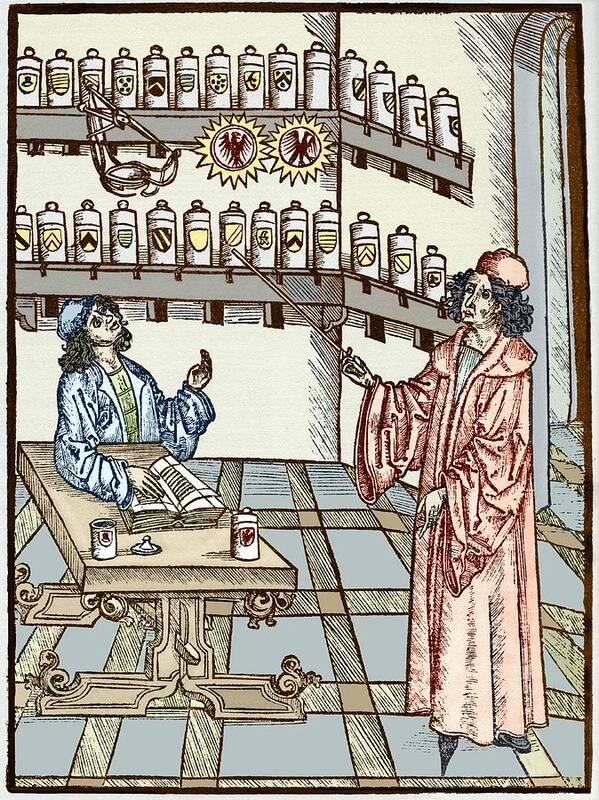The detailed, medieval-style drawing depicts a scene inside an apothecary’s shop, where a teacher in a red robe with pointy black shoes is instructing a pupil. The teacher, standing to the right, is pointing with a long stick towards one of the various ceramic containers on the two shelves mounted on the wall. The containers, some in cylindrical shapes and others with different sizes, hold various substances. The pupil, dressed in a blue robe with a green shirt and blue cap, sits at a wooden desk positioned to the left, with an open book in front of him, looking up attentively at where the teacher is pointing. On the desk beside the book, there are a couple of cylindrical containers. The room's colors are subtle and include pinks, light blues, greens, and light browns. The floor is blue with tan grout, and the perspective on the right side appears slightly off. Notably, there is a scale or cup floating in the air, adding an intriguing element to the scene. The background features an archway behind the teacher, enhancing the vintage, illustrative quality of the artwork.